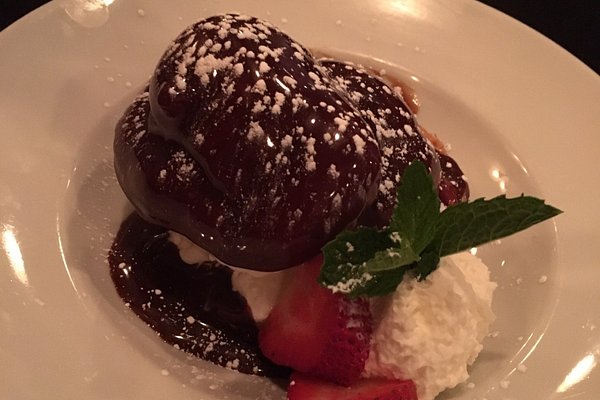A close-up photo captures a delectable pastry adorned with a rich layer of chocolate icing, generously dusted with powdered sugar and sprinkled with petite white sprinkles. The pastry features a prominent cap sitting atop a larger base layer drenched in syrup. Nestled beneath this ensemble is a cushion of white, slightly rough-textured whipped cream, all beautifully presented in a pool of glossy chocolate. Garnishing this sumptuous delight are succulent slices of ripe strawberries and a sprig of fresh mint leaves, adding a pop of color and freshness. The culinary masterpiece is elegantly plated on a pristine white, shallow bowl with a wide rim, set against a completely dark backdrop, highlighting the intricate details and textures.